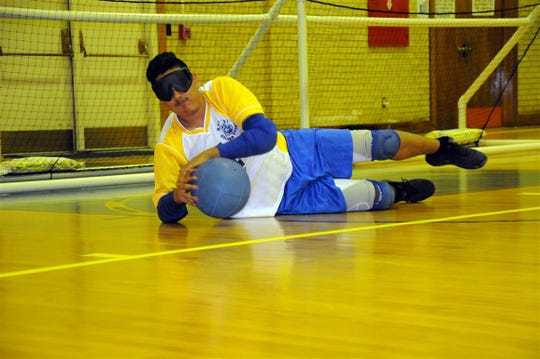The image captures a man in a gymnasium, dressed in a sports uniform comprised of blue knee pads, blue athletic shorts, black shoes, and a yellow and white shirt with blue long sleeves underneath. He is wearing a pair of black ski goggles as blindfolds. The man is positioned near the center of the image, slightly towards the top, and is lying on his right side, propped up on his right arm, clutching a ball that resembles a dodgeball. Behind him, there is a white net extending at an approximate 45-degree angle, and beyond the net, a white brick wall and gymnasium doors with metal push bars are visible. The gym's wooden floor adds to the setting, which is distinctly indoors, with lighting that imbues the scene with a yellowish tint. The color palette in the image includes light brown, off-white, light blue, dark blue, yellow, black, tan, white, red, and orange. Some suggest it might be an action shot of the man either playing indoor volleyball, diving to save the ball, or possibly soccer.